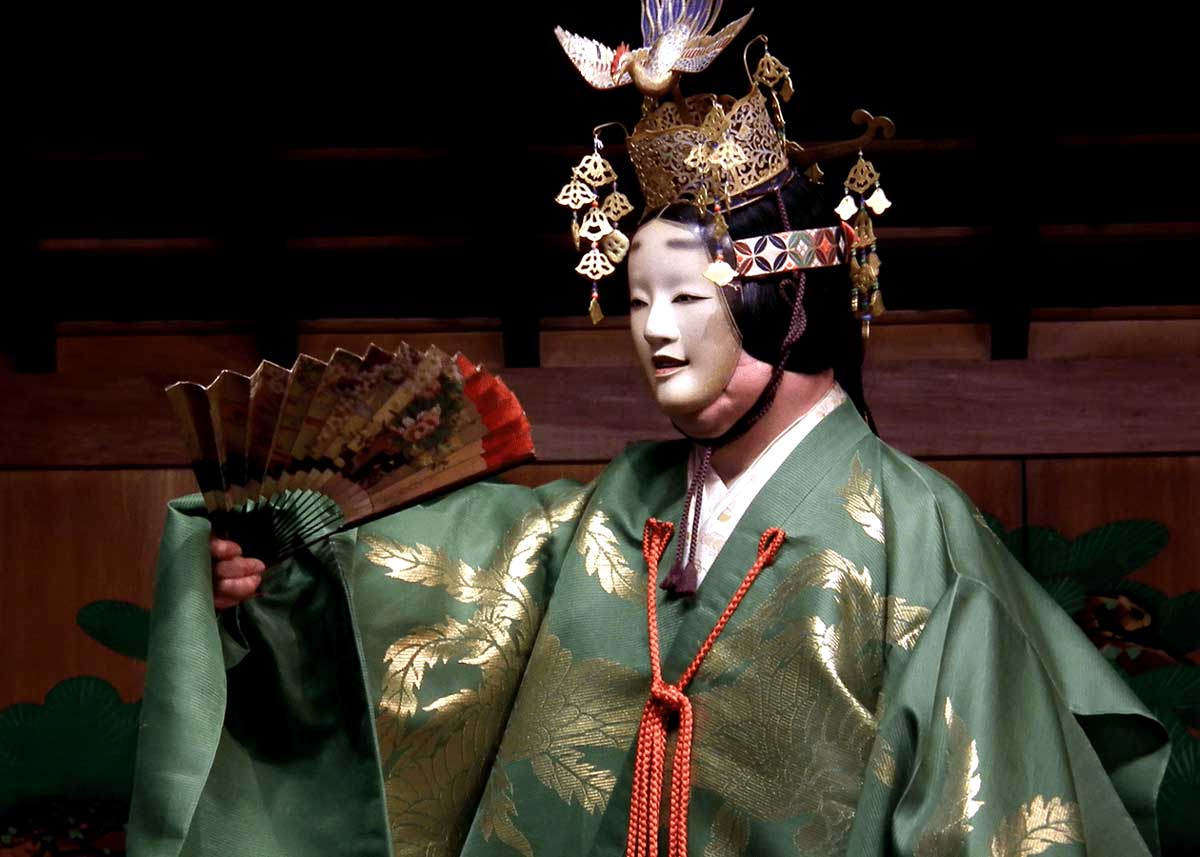The image depicts a kabuki performer standing indoors against a dark, wooden background. The performer is dressed in an elaborate, silk-like, green kimono adorned with gold ferns and secured at the front with a red rope tie. A distinctive white mask with slanted eyes covers the performer's face, complemented by a wig and an ornate headpiece featuring a gold crown with a bird on top and intricate decorations hanging from it. In their right hand, they hold a colorful fan, partially visible as it peeks out from beneath the robe. The setting is dimly lit, casting shadows across the scene, adding to the dramatic atmosphere.